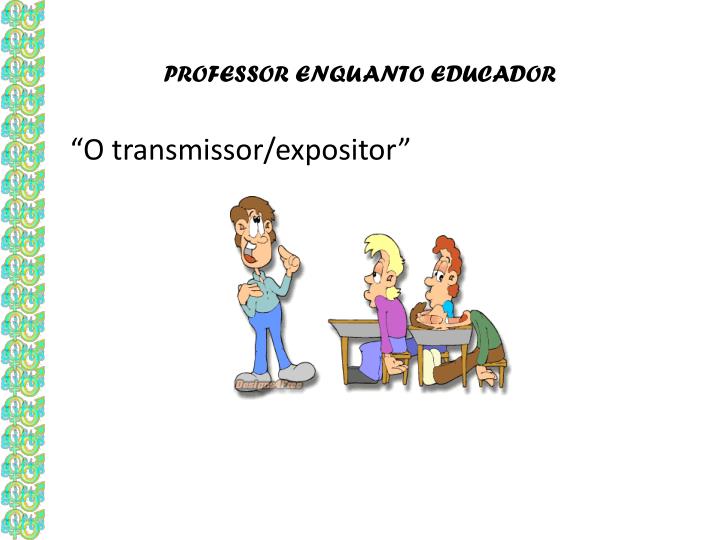In the cartoon image, a teacher stands in front of three students seated at their desks. The scene is framed by a repetitive green border on the left side. The teacher, who has an exasperated expression with his eyes rolling towards the ceiling, is wearing blue pants and gray shoes. Above him, the text "Professor Encuanto Educator" is prominently displayed in bold, with the phrase "O Transmissor/Expositor" underneath it in quotes. 

The students appear disinterested: one male student is asleep with his head down on the desk, another male student, dressed in a purple shirt and violet pants, is looking back towards the sleeping student, and the third student, possibly female, with red hair and a bewildered expression, is staring at the teacher. All characters have exaggerated features such as large heads and long limbs, set against a stark white background, conveying their utter boredom and disengagement with the lesson. The overall composition emphasizes the tedious atmosphere in the classroom and the students' lack of interest in the teacher's lecture.